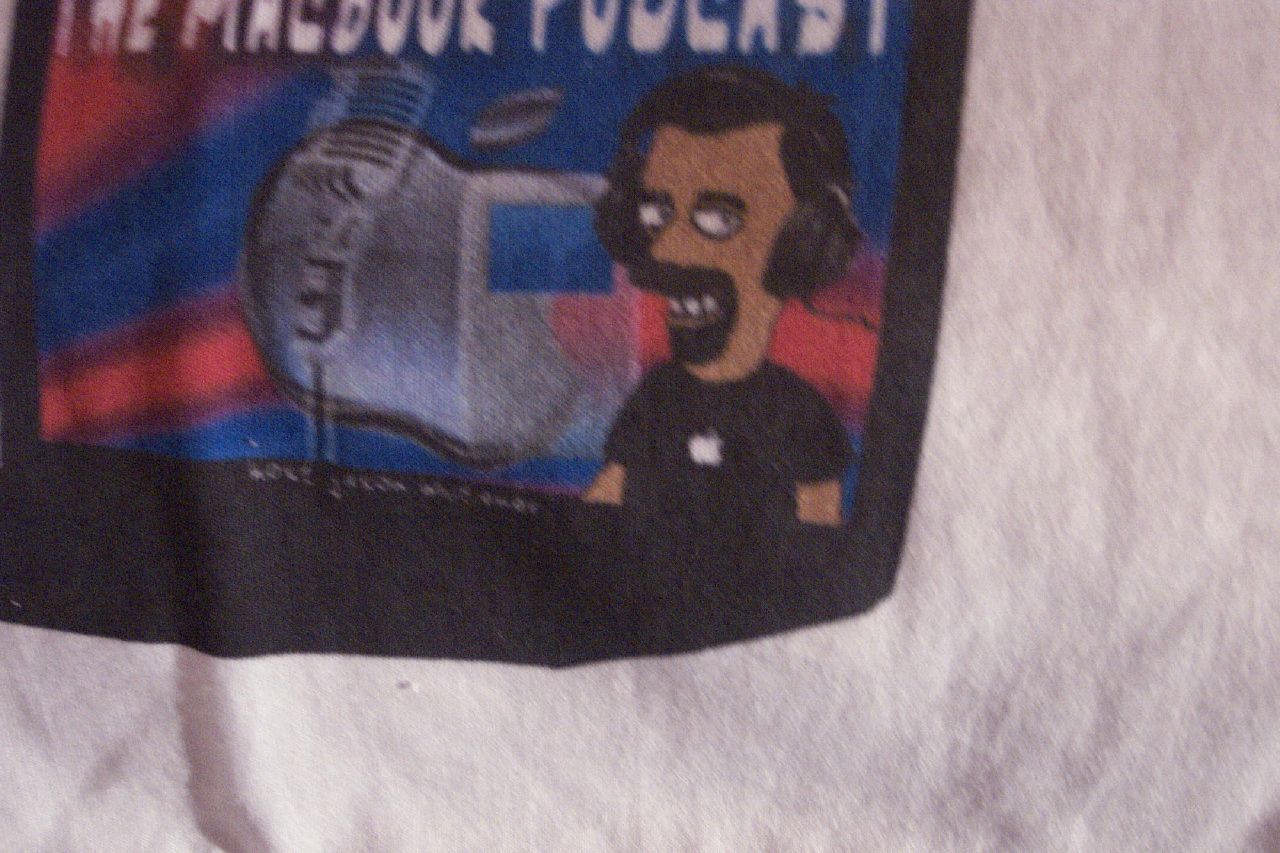The close-up image depicts a printed t-shirt with a white background and a black patch at the center. The patch features a digital illustration of a cartoon-like man resembling a Simpsons character, with dark hair, a full beard, mustache, and goatee, grinning at the viewer. He is wearing wired over-the-ear headphones and a black shirt that has a tilted Apple logo on his chest, which fades out towards the right. Above the man's head, partially cut off but discernible from the visible letters, is the text “The MacBook Podcast.” To his left is an old-fashioned microphone, similar to those used by Elvis Presley, rectangular with lined detailing. The t-shirt also appears slightly wrinkled, enhancing the casual, worn appearance of the fabric.